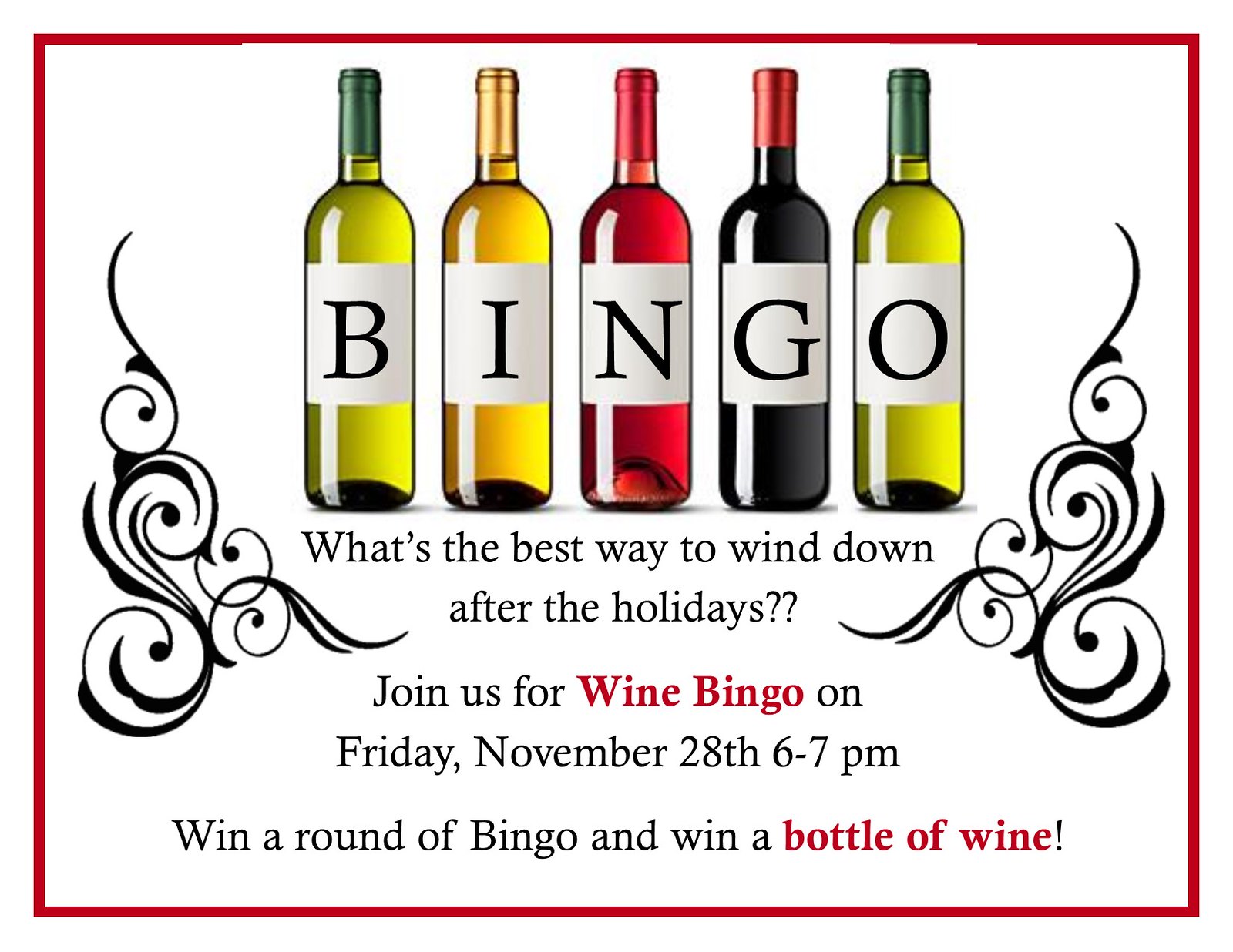This landscape-oriented advertisement is framed by a bold red rectangular border and features a central graphic of five wine bottles in various colors: green, yellow, red, blackish-blue, and green again. Each bottle's white label prominently displays a single black letter, collectively spelling "B-I-N-G-O." Below the bottles, black text asks, "What's the best way to wind down after the holidays?" and announces, "Join us for Wine Bingo on Friday, November 28th, 6 to 7 p.m. Win a round of bingo and win a bottle of wine." The text "Wine Bingo" and "bottle of wine" are highlighted in red. The background is white, and the left and right sides are decorated with black, swirly, embroidered-like borders.